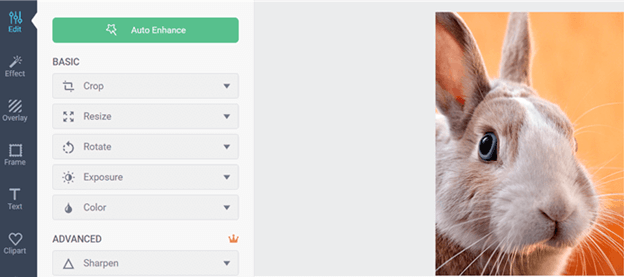Caption: 

The image showcases a photo enhancement website or app interface. On the right side, a user has uploaded a picture of their pet bunny, which features a white and light tan coat, large black and blue eyes, tall tan ears, a prominent bunny nose, and long whiskers. The app provides various controls for photo enhancement. To the left, an "Auto Enhance" button offers a one-click solution to improve lighting and overall photo quality. Basic features such as cropping, resizing, rotating, exposure adjustment, and color adjustment are available for manual edits. Additionally, an advanced menu enables users to sharpen the image for better focus. Other creative options include adding effects, overlays, frames, text, and clip art, making this a comprehensive suite for editing and enhancing photos.